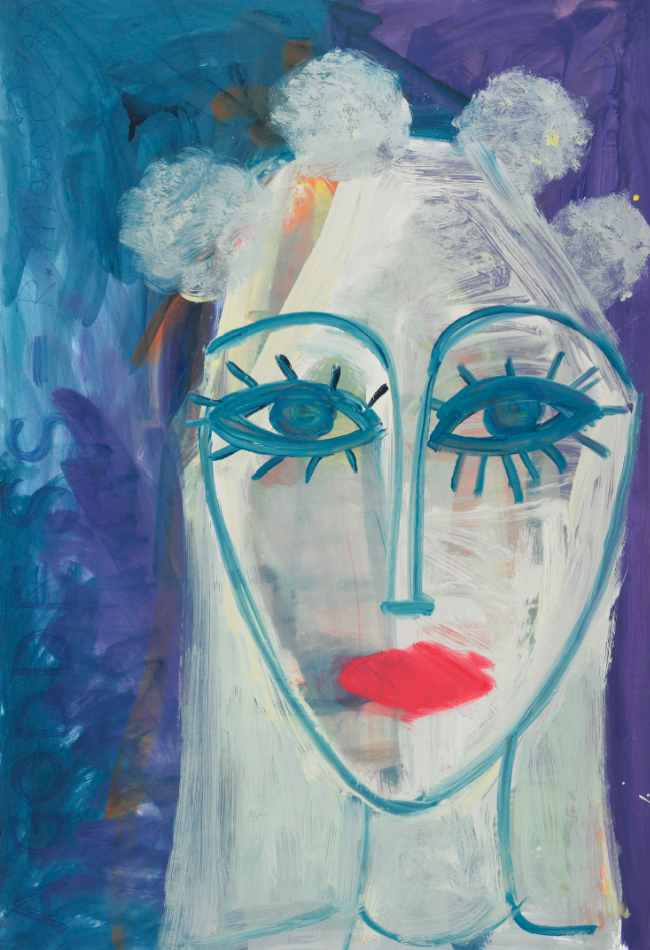The image is a colorful, modernistic drawing of a woman with a heart-shaped, white face and neck. She has strikingly large, dark blue eyes outlined in blue, with emphasized eyelashes radiating like sun rays and very arched eyebrows. Her bright red lips stand out against her white complexion. The woman has a thin, long, and prominent nose. Adorning her head are four spherical, white or crystal-like tufts, possibly resembling a headband or part of her hair, which is straight and white. A yellow streak descends from her forehead towards her right ear. The background gradient transitions from blue to purple. Vertically on the left side, the words "A GODDESS" are written in capital letters, followed by "R. Marcille 89," indicating the artist's signature.